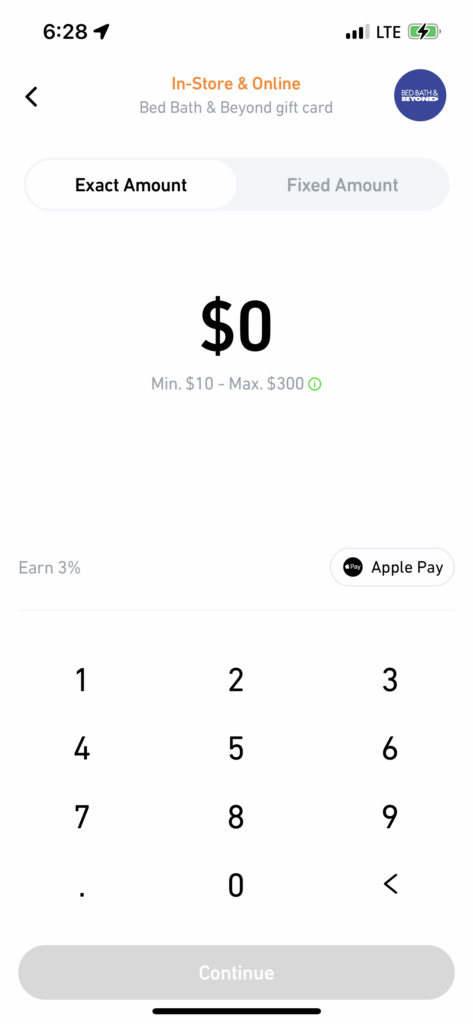The screen of a cell phone is displayed in the image. 

- **Top section:**  
  - **Left corner:** The time is shown as 6:28.
  - **Top right corner:** Indicators for cell signal strength (LTE bars) and a green battery icon indicating charging status.  

- **Main content:**
  - **Upper portion:** 
    - **Left below the top bar:** A left-pointing arrow.
    - **Center:** Text that reads "In-store and online" in orange.
    - **Below the orange text:** "Bed Bath & Beyond Gift Card" in gray. 
    - **Right:** The Bed Bath & Beyond logo within a blue circle.
  
  - **Middle portion:** 
    - Two options: "Exact Amount" and "Fixed Amount". 
      - The "Exact Amount" option is selected.
    - Below "Exact Amount:" It shows "0.00" in black with a dollar sign.
    - Below the amount: "Min $10 - Max $300".
    - Next to this: A green circle containing an 'i' symbol.
    - Below that: "Earn 3%" in gray on the left side.
  
  - **Right side of this section:** A button labeled "Apple Pay".

  - **Lower portion:**
    - **Keypad:** Shows numbers 1 to 9 and 0, arranged in a standard layout.
      - **Left of the keypad:** A dot (".").
      - **Right of the keypad:** A backspace arrow.
    - Below the keypad: A gray button with the text "Continue" in white.
  
- **Bottom part:** A black horizontal band.

The user is attempting to purchase a Bed Bath & Beyond gift card with an exact amount, ranging from $10 to $300, and can earn 3% back for their purchase. The colors used in the design are black, green, gray, white, orange, and blue.